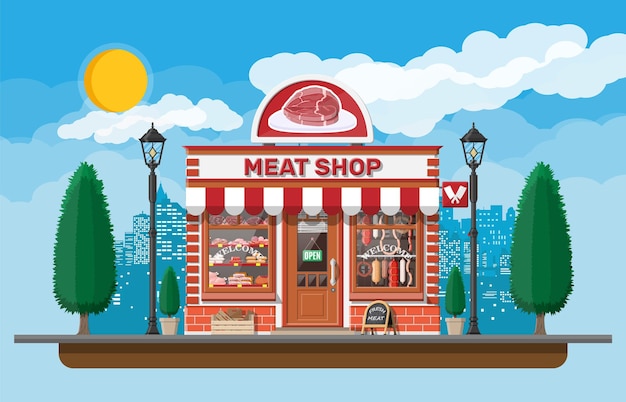The image depicts a digitally-rendered, cartoonish butcher shop made of red bricks, appearing suitable for a game or advertisement. A prominent dome-shaped sign adorning the top of the shop features a white border with a red interior, showcasing a picture of a piece of meat, possibly a ham or steak. Below the sign, "Meat Shop" is written in red, flanked by two crossed meat cleavers. The storefront is detailed with a white and red striped canopy and a visible green "Open" sign on the wooden door. Flanking the door are large glass windows displaying various kinds of meat. On either side of the building, identical black lampposts with diamond-shaped bulbs stand adjacent to pots holding small green trees, which are mirrored by taller trees standing next to the lampposts. The scene is set against a backdrop of a city skyline.